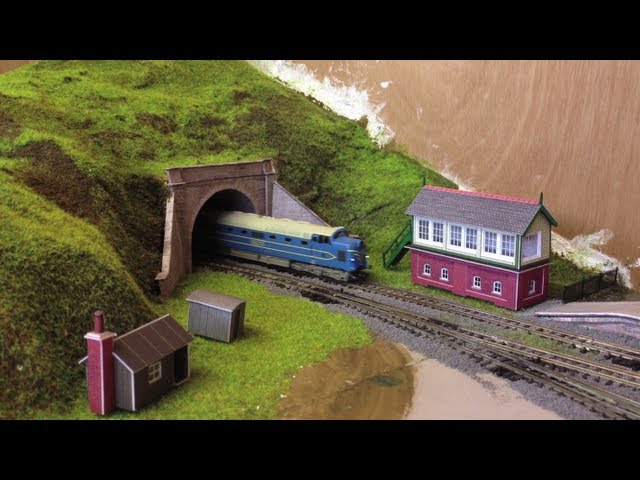This image captures a meticulously detailed model train set. On the left-hand side of the scene, a lush green and mossy hillside stretches across, creating a natural, mountainous landscape. The hillside, adorned with small patches of brown, seamlessly integrates into the scene. Prominently, a tunnel with a brown, shaded entrance emerges from the hillside. Inside the dark tunnel, train tracks extend outward, leading a blue and white locomotive into the scene.

Adjacent to the tunnel, to the left, sits a small house featuring a red chimney stack, contributing to the quaint, picturesque setting. This house is accompanied by an additional small shack, creating a cozy residential feel. The entire left area is a vibrant mix of greenery and model structures, enhancing the scene's realism.

Towards the middle, the model train, a striking blue with a white top, emerges from the tunnel, positioned on realistic-looking train tracks. As your gaze follows the train to the right-hand side of the scene, a two-story building comes into view. The lower floor of this building is red with four windows, while the upper floor is white featuring six windows and one large window around the corner, capped with a gray roof. This building, potentially residential or professional, stands near a brown, wall-like structure that could be wooden and provides a backdrop for the entire intricate model.

Overall, the detailed craftsmanship of the model train set, with its varied landscapes and structures, creates an engaging and lifelike diorama, devoid of any signages or signatures, allowing the viewers to immerse themselves in the miniature world.